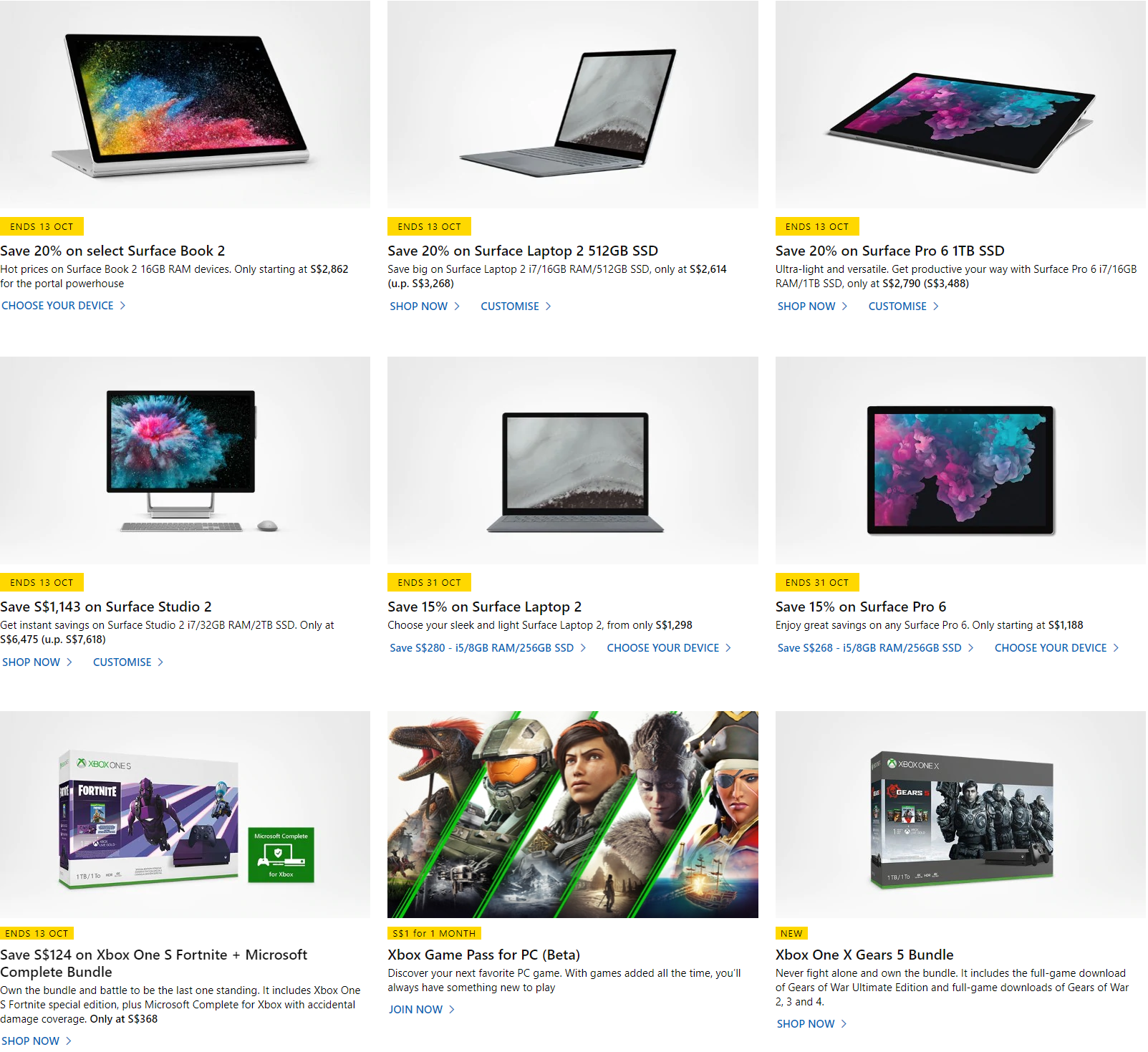This image is a screenshot from a shopping website featuring a grid layout of nine electronic products available for purchase, each arranged in three rows and three columns. The products are displayed with significant discounts and end dates for the offers highlighted in yellow text beneath each item. 

**Top Row (Left to Right):**
1. Save 20% on select Surface Book 2.
2. Save 20% on Surface Laptop 2 with a 512GB SSD.
3. Save 20% on Surface Pro 6 with 1TB SSD.

**Middle Row (Left to Right):**
1. Save $1,143 on Surface Go 2.
2. Save 15% on Surface Laptop 2.
3. Save 15% on Surface Pro 6.

**Bottom Row (Left to Right):**
1. Save $124 on Xbox One S Fortnite + Microsoft Complete Bundle.
2. Xbox Game Pass for PC.
3. Xbox One Gears 5 Bundle.

All promotional offers are prominently displayed, and it is noted that most of these deals end on October 13th. The precise end dates are indicated in yellow text directly under each product listing.